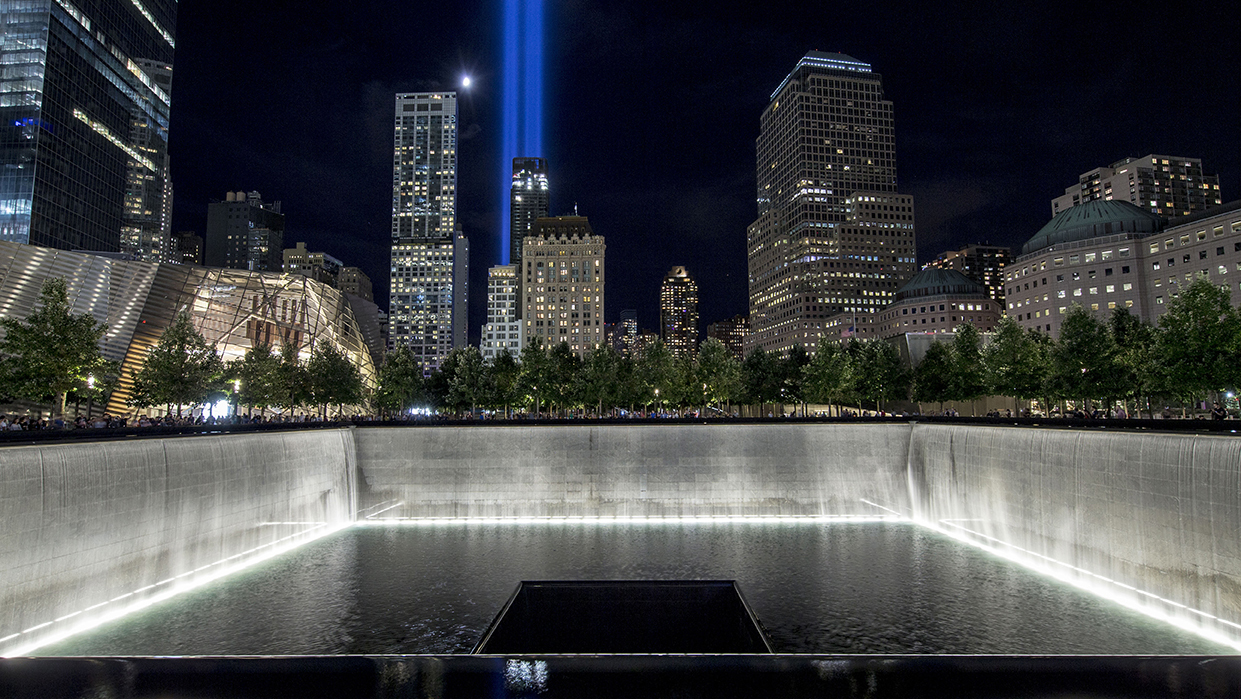The image captures a stunning night view of a city's skyline, most likely New York, from the vantage point of a large, square-shaped fountain or pool. The illuminated pool is surrounded by a line of triangular green trees, creating a lush barrier against the backdrop of the city's skyscrapers. The buildings vary in size and design, with notable features including a tall structure with two green domes and another with a distinctive rectangular brace. The dark, starless sky enhances the brilliance of the city's lights, with windows of the lit skyscrapers sharply highlighted. Dominating the scene are two bright blue light beams reaching skyward, reminiscent of the tribute lights near where the One World Trade Center once stood. The moonlight hovers close to these beams, adding to the enchanting nighttime atmosphere.